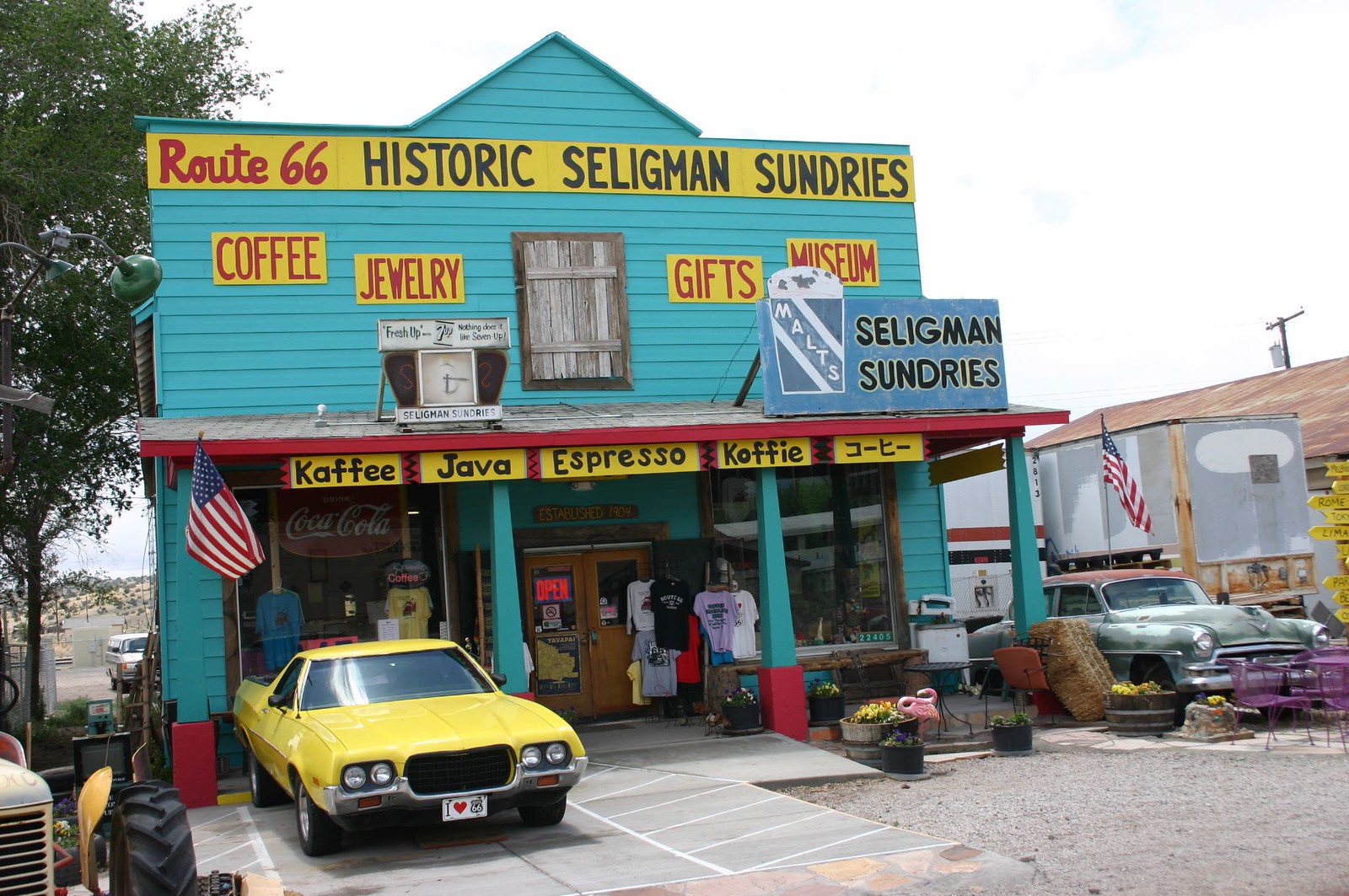The photograph captures an eclectic and historic storefront of the Seligman Sundries on Route 66. The old-fashioned rectangular building is painted a distinct blue with contrasting red trim and a grey roof. Prominent yellow signs adorn the facade, detailing various offerings with red lettering: "Coffee," "Jewelry," "Gifts," and "Museum." At the top, larger signs proclaim "Route 66" in red text and "Historic Seligman Sundries" in black text, creating a vintage and nostalgic feel.

The parking lot in front features two notable vehicles: a polished, old-fashioned yellow muscle car, and a rusting silver car from the 1950s. Additional details around the storefront include a blue sign reading "Maltes Seligman Sundries," various unique displays such as whiskey barrels filled with flowers, an antique washing machine by the window, a tree stand with t-shirts for sale, and signs pointing to distant destinations like Rome.

Further adding to the character, the store's windows and entrance are peppered with vintage decor including a Coca-Cola sign and an American flag mounted near the door. The front door itself is wooden with glass inserts, welcoming visitors into this charming slice of Americana.